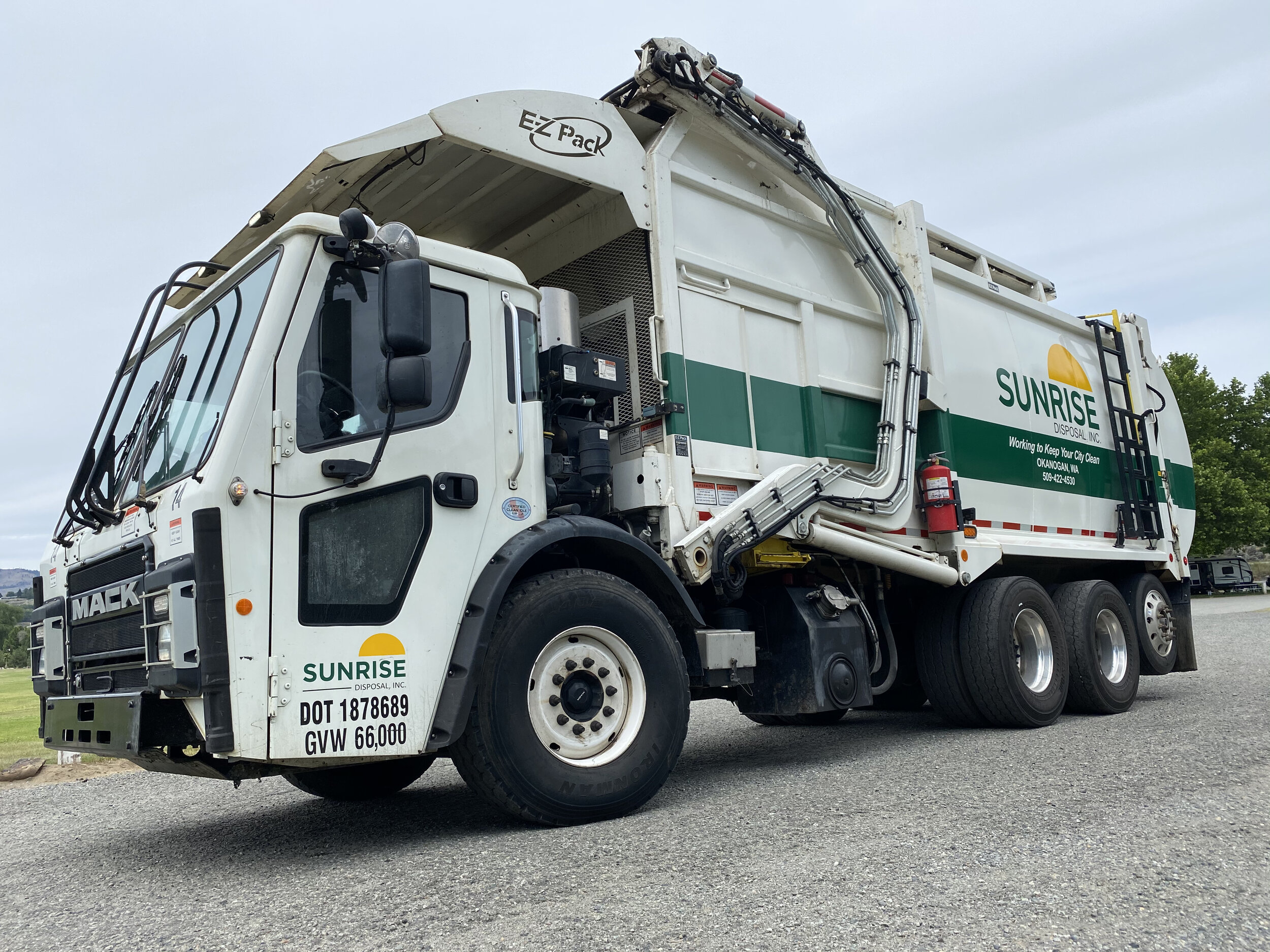This image depicts a large white Mack garbage truck with a green stripe along its side, prominently displaying the logo and text "Sunrise Disposal Incorporated" and the motto "working to keep your city clean". The location mentioned is Okanagan, Washington. Positioned on a gray concrete driveway, the truck's front and one side are visible in the frame. Notably, the side and driver's door include various identification numbers: a somewhat illegible phone number, a Department of Transportation (DOT) number (18786689GVW6600), and the label "EZ-Pack" atop the trash compactor. The truck, possibly with 18 wheels, dominates the visual space, leaving only glimpses of green lawns, trees with green leaves, and a streaked gray sky in the background. The asphalt surface beneath the truck adds to the overall gray ambiance of the scene.